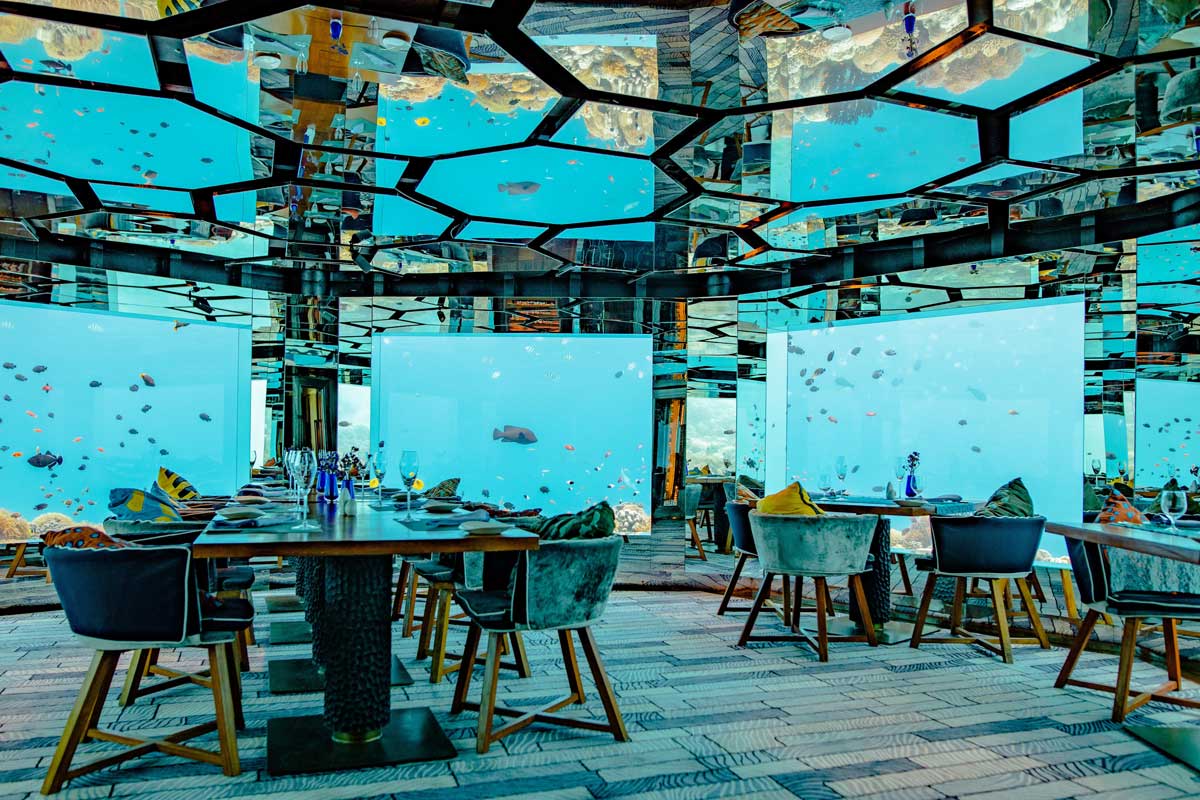The image depicts a detailed artwork or painting of an underwater restaurant, enclosed within a glass structure that allows for breathtaking views of the surrounding ocean. The restaurant’s interior features a series of reflective tables and chairs arranged in an inviting manner, with the first set located on the left and another set positioned on the right. The tables appear to be made of a glossy material, reflecting the aquatic environment outside. The ceiling is adorned with a striking pattern of hexagons and squares, also reflective, mirroring the vibrant scene below. The rich color palette includes various shades of blue, from dark to light, intermixed with yellows and blacks.

Adding to the mesmerizing ambiance, the walls of the restaurant display multiple screens that project dynamic underwater scenes, showcasing schools of fish and vibrant coral reefs. These images, coupled with the actual view through the glass panes, create an immersive experience, making diners feel as though they are truly part of the ocean. Fish swim gracefully around the enclosure, enhancing the illusion of the underwater setting and contributing to the restaurant's unique and enchanting atmosphere.